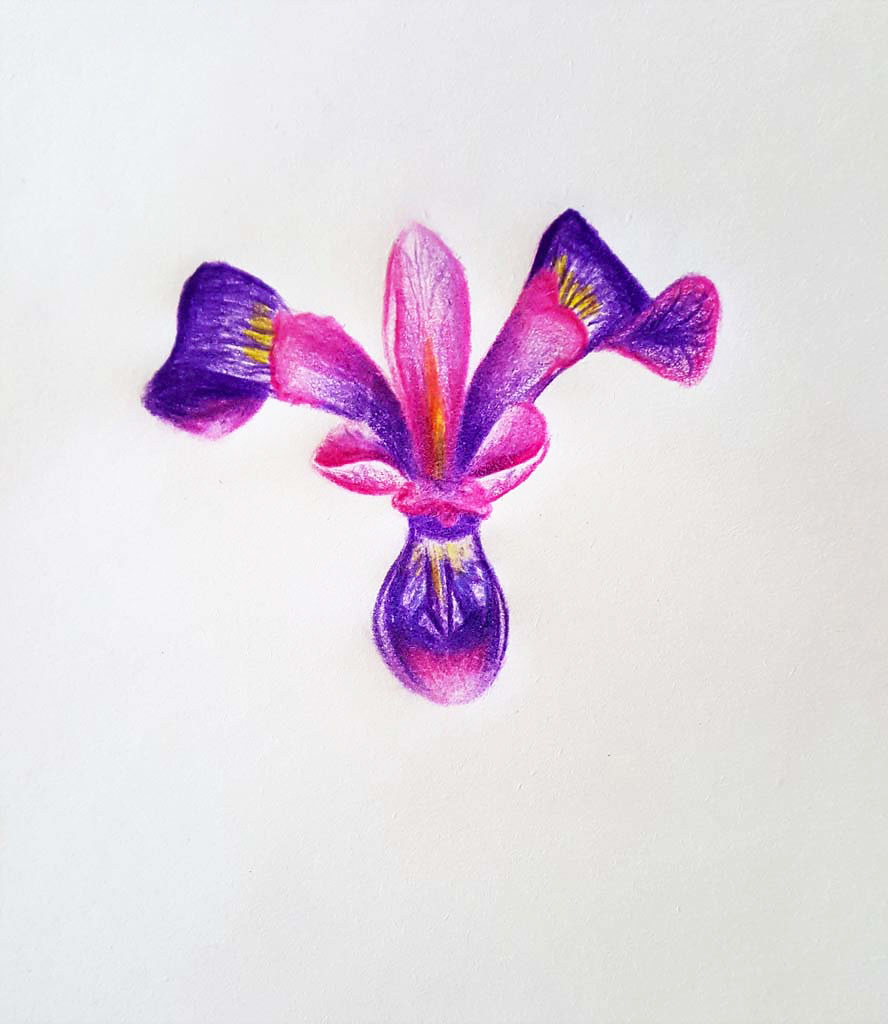This detailed crayon illustration on a white piece of paper features a uniquely designed flower. The flower's base is notably rounded and bulbous, creating a solid foundation for the sprawling petal arrangement. The central petal extends straight upward, flanked by additional petals that arch outward, one to the left and one to the right, with small gaps separating them. Closer to the base, a couple of petals emerge, completing the dimensional and lively composition. The predominant colors are rich shades of purple and blue, with subtle accents of yellow adorning the tips of some petals, adding a delicate contrast and enhancing the visual interest of the artwork.